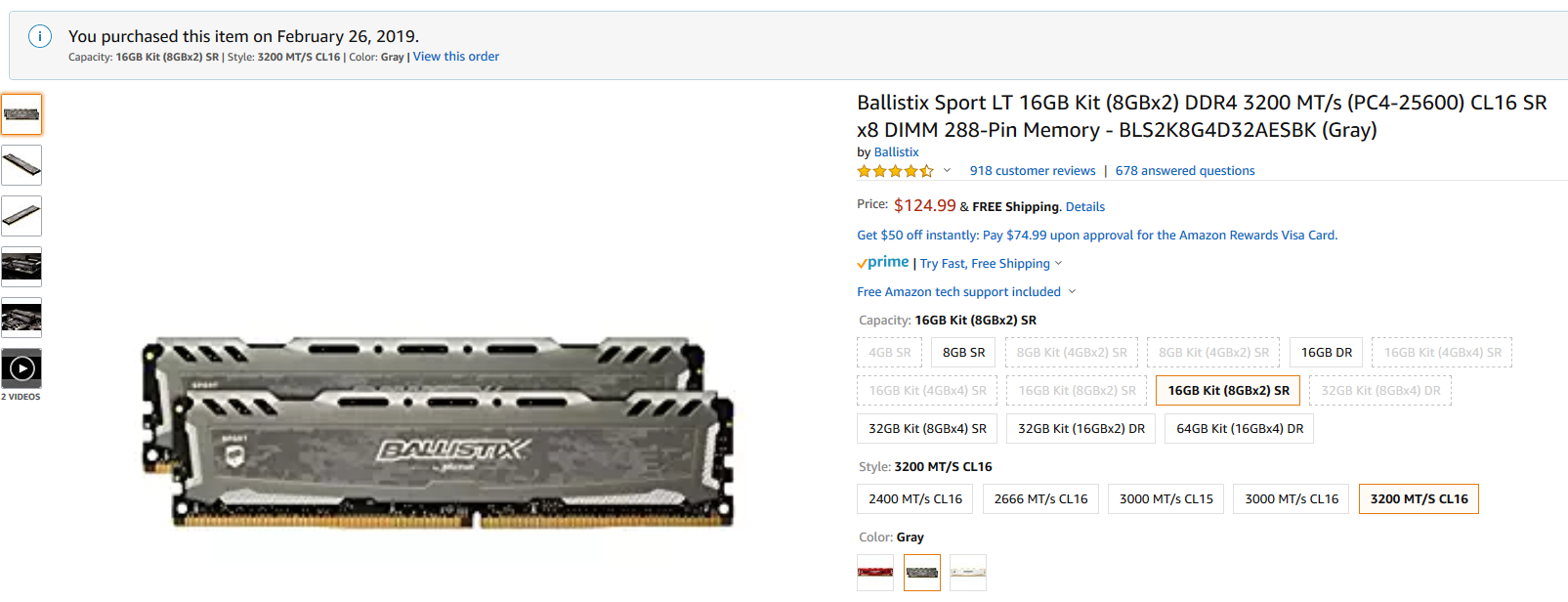This is an image depicting a screenshot of a computer screen showing an Amazon shopping page. At the very top, there's a light gray toolbar stretching across the screen, featuring a small circle with an 'i' icon. The icon is accompanied by the message, "You purchased this item on February 26, 2019."

The left side of the screen showcases a large image, possibly of a computer hardware component. The component appears to be a set of memory sticks, often described as ball sticks, with a gray color scheme, suggesting they might be vehicle parts or, more likely, computer memory modules. Below this main image, there are six smaller thumbnail images. The top thumbnail is highlighted with a yellow border, indicating it is the currently selected image. The bottom thumbnail features an emblem for a video with a play button in a circle.

On the right side of the screen, there's a detailed product description. The text reads: "Ballistix for an LT 116, 16GB Kit (8GBx2) DDR4-3200 MT/s (PC4-25600) CL16 SR x8 DIMM 288-Pin Memory." Additionally, there is a part number listed, though not fully detailed in the caption. The item is priced at $124.99, with the price displayed in red.

Below the price, there appears to be more information, potentially offering an option to select different sizes or specifications of the product.